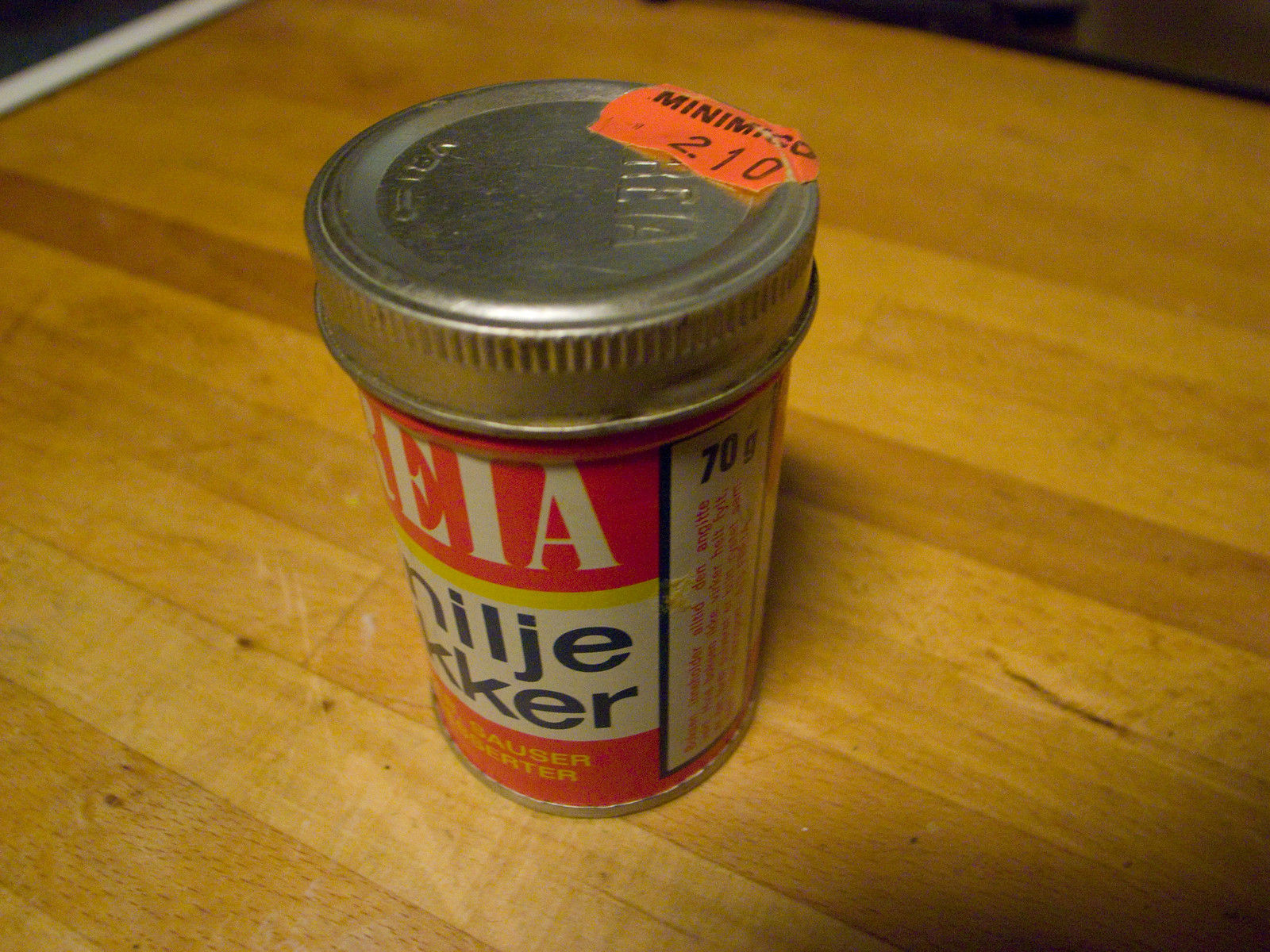In the photograph, a small silver metal canister with a lid is situated on a worn wooden surface. The wood, characterized by its light orangey-beige hue, displays signs of use with scuffs and dents marring its appearance. The background, captured behind the wooden surface, is a nondescript dark gray, adding a stark contrast to the scene.

The cylindrical canister features a silver lid adorned with a price tag sticker indicating a cost of $2.10. Wrapping around the body of the canister is a red label, distinguished by a white patch in its center. Prominent white letters at the top of the red label spell out "EIA." Within the white patch, the words "NILJE KKER" are inscribed in navy blue letters. Below this, additional text can be seen, though it is less legible and appears in yellow on a red background.